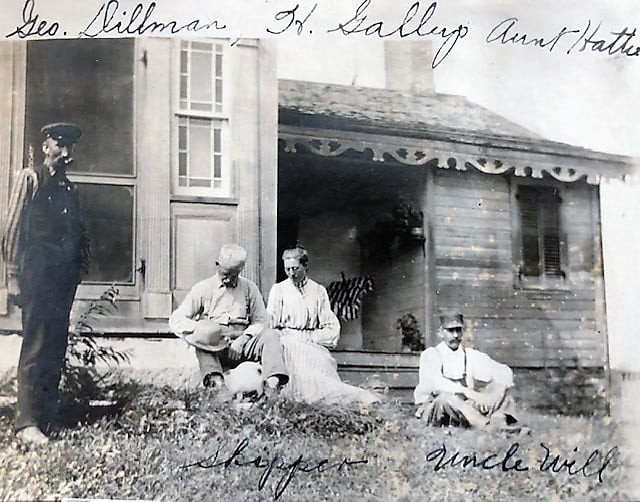This large, square black-and-white photograph appears to be from the early days of photography, depicting a group of four people in front of a rundown wooden house with horizontal slats. The cloudy sky above hints at an overcast day. Handwritten in black ink at the top of the image are the names "Geo Dillman H Gallop Aunt Hattie." 

The house, showing signs of age and wear, features a front porch accessed by a few wooden steps. Sitting on these steps in the center of the photo are two older individuals—an elderly man with a hat resting on his knee and looking down, and an elderly woman in a long white dress, gazing downwards towards him. 

To the right of this couple, another man sits on the grass, with his elbows on his knees, staring ahead. Handwritten beneath him is the name "Uncle Will." On the left side of the image, a man stands in front of a window. He is dressed in some sort of uniform with a black hat, potentially indicating he may be a police officer. Each person’s attire adds a sense of historical context, reflecting their fashion from a bygone era. The photograph captures not only the individuals but also a glimpse into their lives, emphasizing the simplicity and austerity of their surroundings.